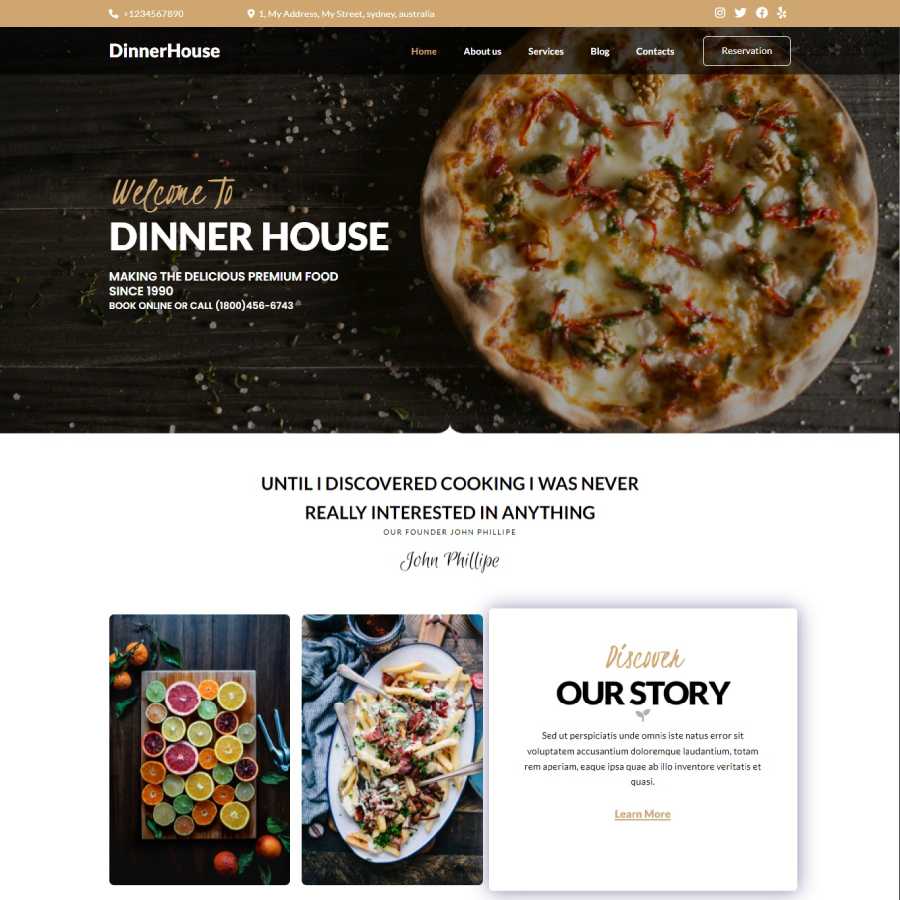The image showcases the homepage of "Dinner House" restaurant's website. At the top of the page, a contact number, location details, and social media icons for Instagram, Twitter, and Facebook are prominently displayed. The navigation menu features tabs for Home, About Us, Services, Blog, Contact, and Reservation, with the Home tab visually highlighted in brown, while the others remain white.

Centrally positioned, the text "Welcome to Dinner House, making delicious premium food since 1990. Book online or call 1800-456-6743" invites visitors to engage with the restaurant. To the right of this welcoming message, a mouth-watering image of a brown pizza on a dark brown table, complete with pizza crumbs, serves as the background, enticing potential customers.

Beneath the inviting message, a quote reads, "Until I discovered cooking, I was never really interested in anything." This is attributed to the restaurant's founder, John Filipe, whose name is elegantly signed in black text.

At the bottom right corner, a prompt "Discover our store" hints at more offerings, with an unspecified date written in a foreign language and a brown "Learn more" button encouraging further exploration.

On the left side of the image, photographs of fresh ingredients like onions, oranges, blood oranges, nachos, and green lemons are displayed on a chopping board. Adjacent to this is a white plate containing three silver spoons, each filled with food, adding to the overall culinary appeal.